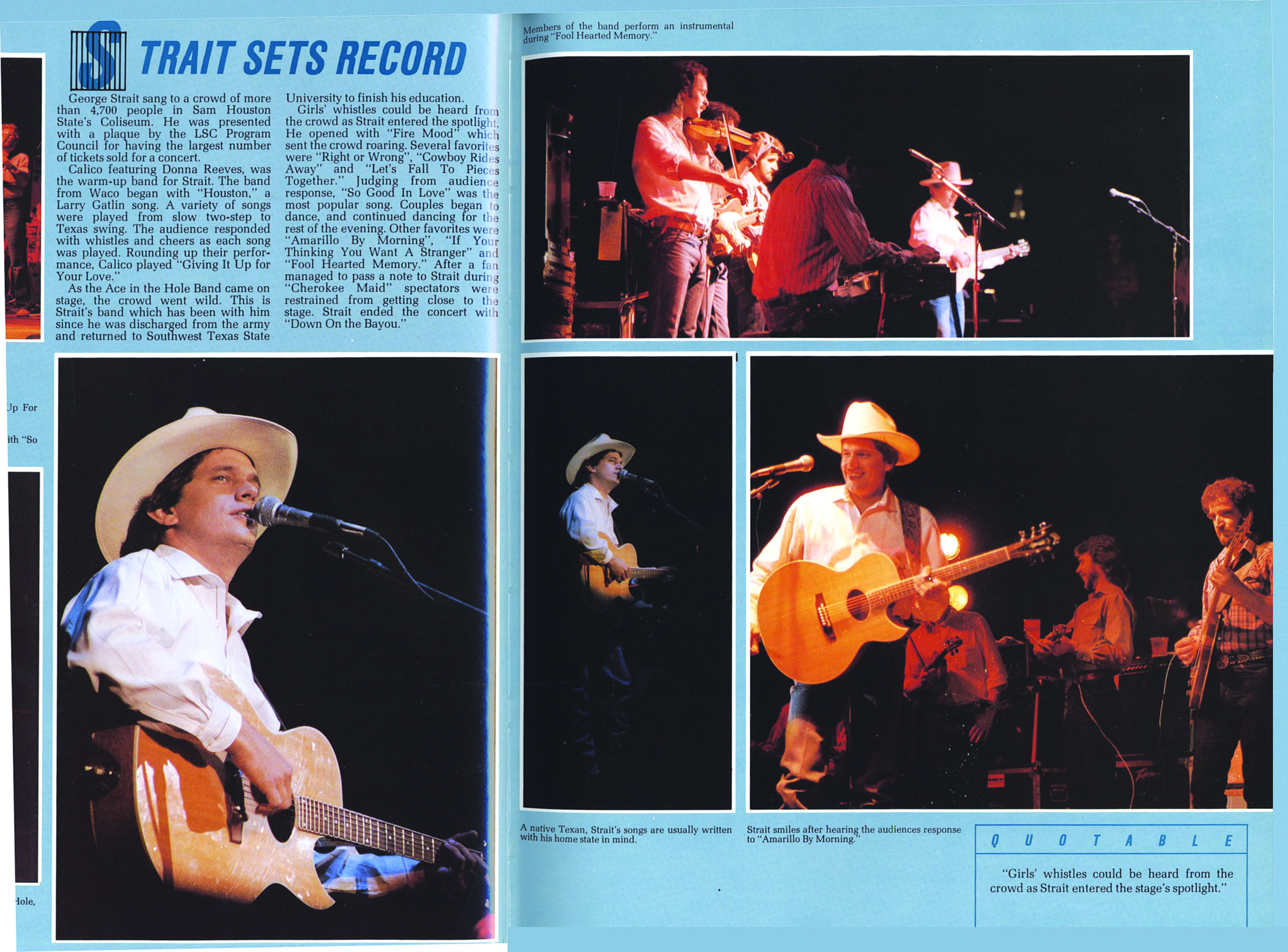This image captures an article about country music singer George Strait, presented in a two-page magazine format with a light blue background. The heading "Strait Sets Record" appears in the upper left-hand corner in dark blue text. The article details George Strait's performance to a record-breaking crowd of over 4,700 people at Sam Houston State's Coliseum, where he was honored with a plaque by the LSC Program Council for achieving the highest number of tickets sold for a concert.

On the left page, a prominent photograph of George Strait against a black background features him seated and playing an acoustic guitar, wearing a white cowboy hat, a white collared shirt, and singing into a microphone positioned to the right of the image. 

To the right, a page filled with images showcases three distinct photographs: one large, vertical close-up of Strait singing into a microphone, and two larger horizontal images. The first horizontal image portrays George Strait performing solo, while the second features him alongside his entire band, with Strait standing prominently in the front left. At the bottom right corner of this page, a section labeled "quotable" contains black text stating, "Girls' whistles could be heard from the crowd as Strait entered the stage's spotlight."